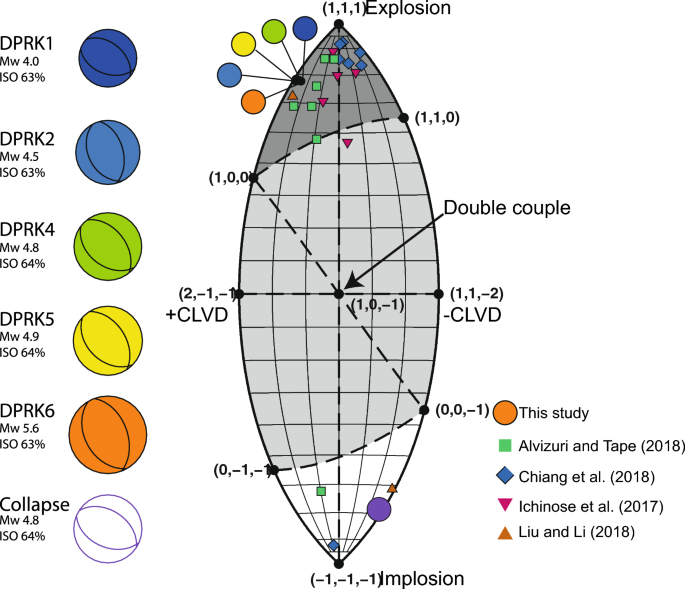The image depicts a scientific diagram that combines multiple datasets related to explosion and implosion events. On the left side, there are six circular data points resembling basketballs with spherical lines through them, each labeled with DPRK and COLLAPSE event names, isotopic percentages, and magnitudes such as DPRK1MW4ISO63, DPRK2MW4.5ISO63, DPRK4MW4.8ISO64, DPRK5MW4.9ISO64, DPRK6MW5.6ISO63, and COLLAPSEMW4.8ISO64. The circles are color-coded: dark blue, light blue, green, yellow, orange, and white with a purple outline respectively. These circles correspond to different studies—orange for this study, green for Al-Waziri and Tape, blue for Chang, pink for Itanus et al., and an orange triangle for Lu and Li.

The central graph has an almond or blimp shape, with an explosion labeled at the top and implosion at the bottom, with various data points and labels, including a central "double couple." Arrows and dashed lines indicate relationships and data trajectories. The diagram provides a comprehensive, multi-source visualization of the seismic events analyzed within these studies.